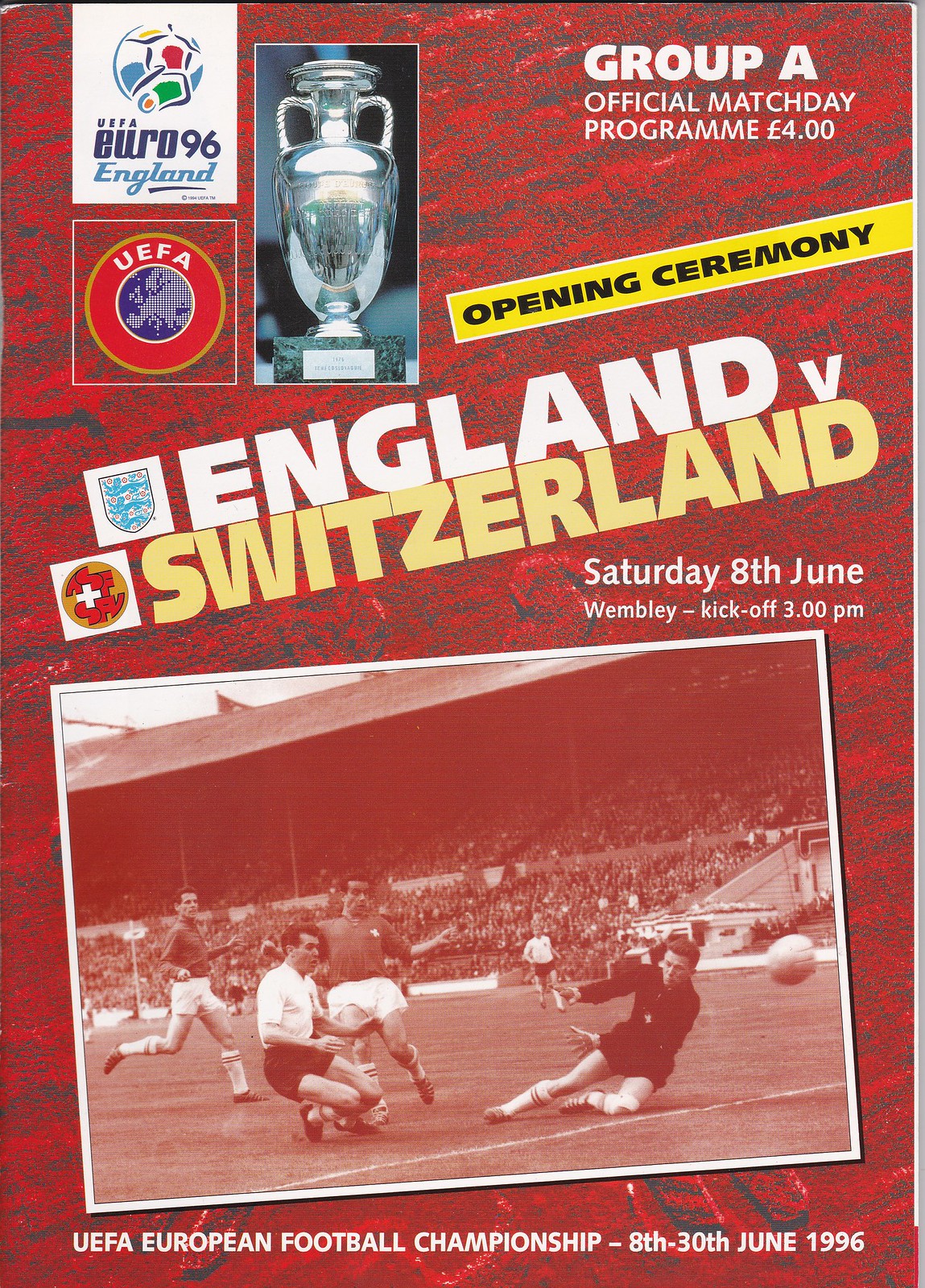The image is a vertically aligned, full-color cover of a program or magazine for a historic soccer match. The background features a blend of red and gray, textured to resemble wood with cloud-like patterns at the top. In the upper left corner, a white box displays the Euro 96 England logo with a soccer ball image and "UEFA" beneath it, framed by a white square. To the right, there's a black and white photograph of a silver trophy. The upper right corner prominently states "Group A" in bold, white letters, followed by "Official Match Day Program 4.00" in black print on a yellow rectangle. Diagonally across the middle, large white letters spell out "England V Switzerland," with "Switzerland" displayed in light brown. Below this, it states, "Saturday 8th June Wembley kickoff 3 p.m."

The center of the cover features a sepia-toned photograph showing a lively soccer match with players in vintage attire, a dynamically flying soccer ball, and packed stands in the background. This image is framed by a white border. At the bottom, in white text, it reads, "UEFA European Football Championship 8th-30th June 1996."